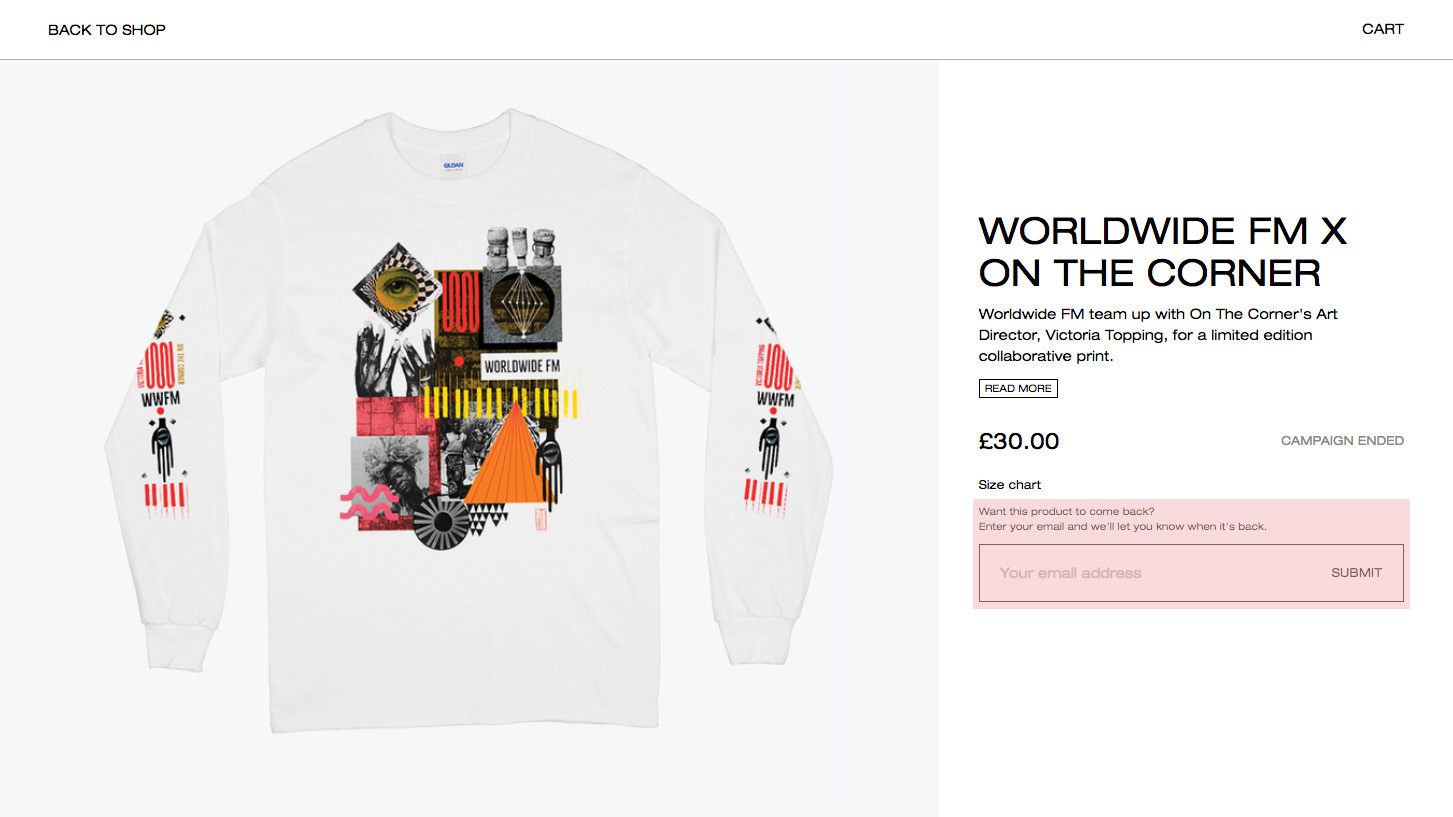This image is a detailed screenshot from a shopping website, featuring a white-background interface. In the upper left corner, there is a "Back to Shop" link in black font, while the upper right corner displays a "Cart" link. Below this, a horizontal black line separates the header from the main content.

On the left side of the screenshot, there is an off-white backdrop showcasing a white long-sleeved t-shirt adorned with various graphics. The chest area of the t-shirt features a square-shaped collage, including an eye, geometric designs, and an image of a Black woman with an afro. Additionally, the sleeves are decorated with the text "WMFM," along with graphics of a hand and a piano.

On the right side of the image, bold black font reads "Worldwide FMX" in the upper corner. Below this, a detailed description states: "Worldwide FM teams up with Art Director Victoria Topping for a limited edition collaborative print." Immediately beneath this text is a "Read More" button, followed by the price of "£30". To the right of the price, in gray font, it indicates that the "Campaign Ended".